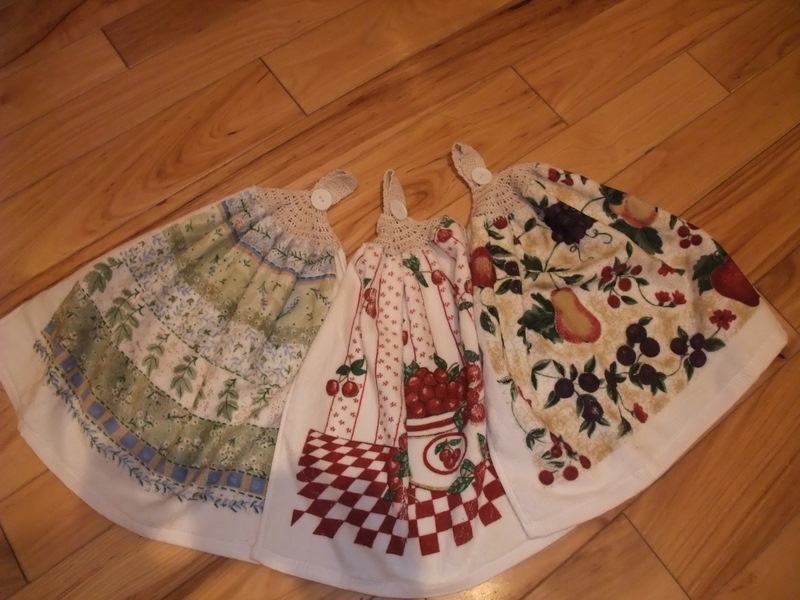The image depicts an aerial view of three terry cloth kitchen towels laid out on a light brown, wood vinyl floor with thin planks that have a reddish tint and visible grain lines. Each towel features a handcrafted knitted top section with a beige button and a loop for hanging.

1. The first towel has an off-white beige background adorned with blue and green leaves, tiny flowers, and a beige knitted top.
2. The second towel displays a red and white checkered pattern, centered around a white ceramic vase filled with cherries, complemented by additional scattered cherries and red dots against a white background. It also has a beige knitted top.
3. The third towel showcases a beige background with green leafy vines featuring orange-colored fruits resembling peaches or mangoes, along with small red accents that could be berries or flowers, paired with a beige knitted top.

These towels evoke a nostalgic, handmade feel, reminiscent of those common in Midwest kitchens during the 90s.